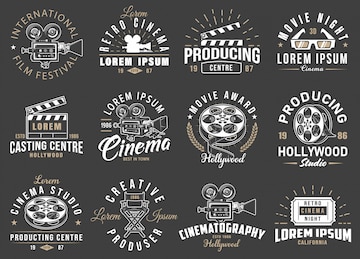The image features 12 distinct logos for various film-related organizations, arrayed in a grid of four across and three down. Each logo is designed in either light tan or white against a dark gray to black background. The text on these logos includes names like International Film Festival, Retro Cinema, Producing Center, Movie Night, Casting Center, Cinema Studio Producing Center, Creative Producer, Cinematography, and multiple instances of "Lorem Ipsum." Additional graphical elements include classic Hollywood iconography such as an old-fashioned camera with spinning movie reels, the clapperboard used in film production, a movie film reel, and a movie ticket. These elements combine to create a cohesive representation of diverse film industry entities, unified by a consistent color scheme and thematic imagery.